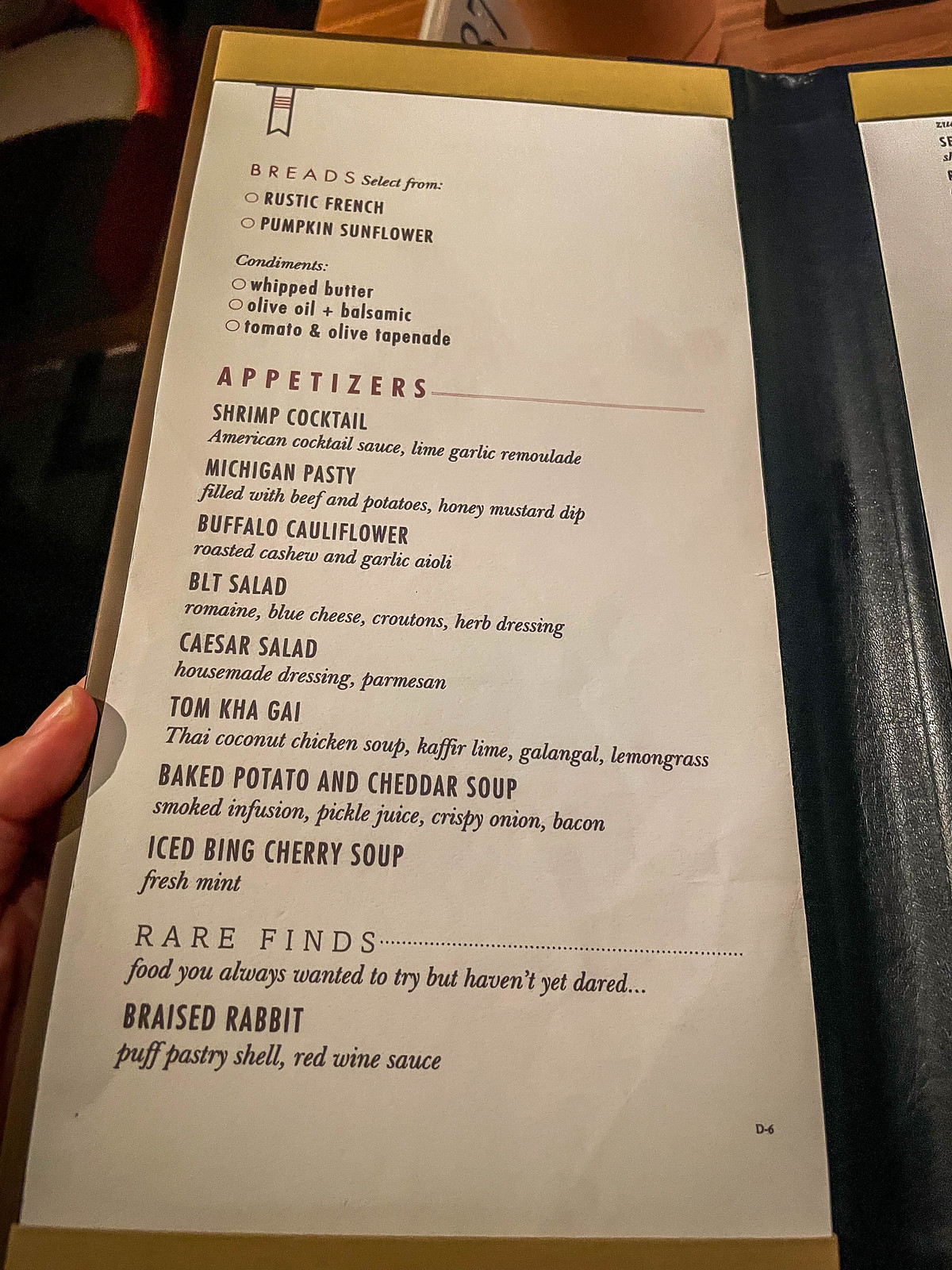The image features a close-up of an individual's hand, revealing only their finger, holding an elegantly designed black leather menu. The finger, suggesting a person of fair complexion, delicately supports the menu, emphasizing its high-end appearance. 

The visible left side of the menu indicates it is part of a two-fold design. At the top, the heading reads "Breads," under which patrons are invited to "select from" an assortment of breads including Rustic French and Pumpkin Sunflower. Additionally, a selection of condiments such as whipped butter, olive oil, balsamic tomato, and olives is listed.

Below the bread section, a list of appetizers is featured. Options include:

- Shrimp Cocktail with garlic
- Michigan Pasty
- Buffalo Cauliflower
- BLT Salad
- Caesar Salad
- Tom Kha Gai, described as a Thai coconut chicken soup
- Baked Potato and Cheddar Soup
- Iced Bing Cherry Soup

At the very bottom of the menu, there is a section titled "Rare Finds: Foods You Always Wanted to Try but Haven't Yet Dared," highlighting a unique offering of braised rabbit.

The detailed layout of the menu, along with the upscale leathery texture, suggests a sophisticated dining experience.